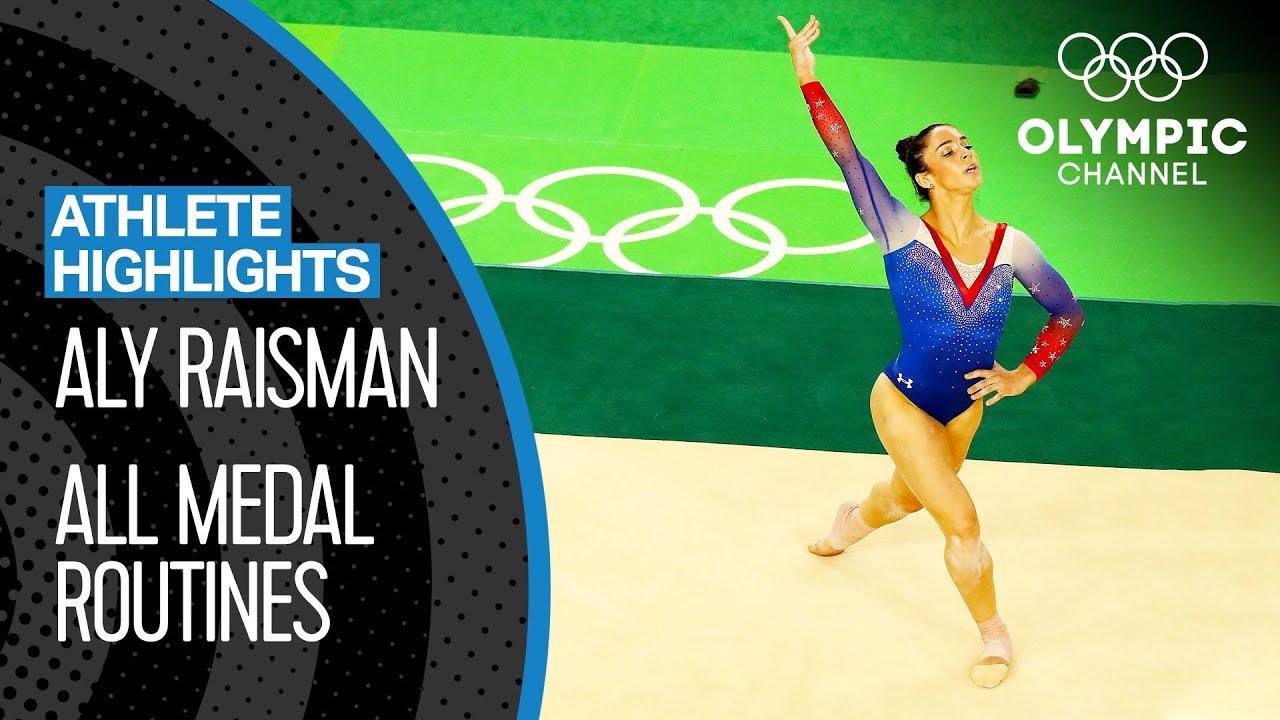The image is an advertisement for the Olympic Channel, prominently featuring American gymnast Aly Raisman. In the upper right corner, the iconic Olympic rings are displayed in white with the text "Olympic Channel" beneath them. Aly is shown in an athletic pose, dressed in a red, white, and blue leotard, which reflects the colors of the American flag. She stands on a tan mat with aesthetic tape on her feet, her left hand placed on her hip, and her right hand extended high above her head. Behind her, the Olympic rings are visible on the ground. To the left, a section of the image highlights her achievements: it reads "Athlete Highlights" against a blue background, with "Aly Raisman" and "All Medal Routines" in white text. The overall background is green with a darker green stripe running through the middle, and a semi-circle display emphasizes the athlete highlights, framed in black and gray with a blue outer rim. The image captures both the athletic prowess and the patriotic spirit associated with the Olympic Games.